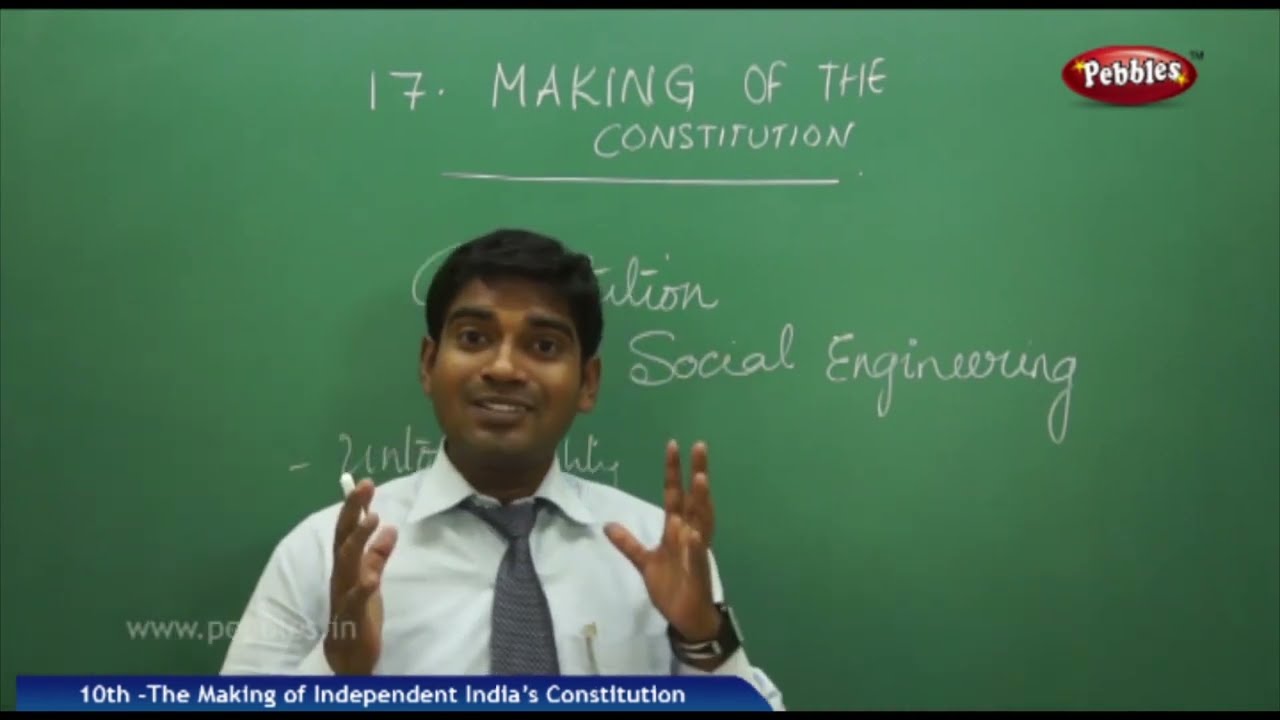The image appears to be a screenshot of a classroom setting, capturing a moment where a man, likely a professor, stands in front of a green chalkboard. The professor, who has black hair and appears to be of Indian descent, is dressed in a white button-down shirt with a tie and is holding a piece of chalk. He also wears a watch. He seems to be in the middle of teaching, with his hands raised and a slight smile, possibly in the process of explaining something.

On the chalkboard behind him, prominently written in white chalk, is "17, Making of the Constitution" which is underlined, and beneath that "Social Engineering." The man is partially obstructing some additional text on the board. The image has thin black bars across the top and bottom. In the upper right-hand corner, there is an oval red icon with the word "pebbles" written in white font. At the bottom left of the image, a blue banner with white lettering states, "10th, The Making of Independent India's Constitution."